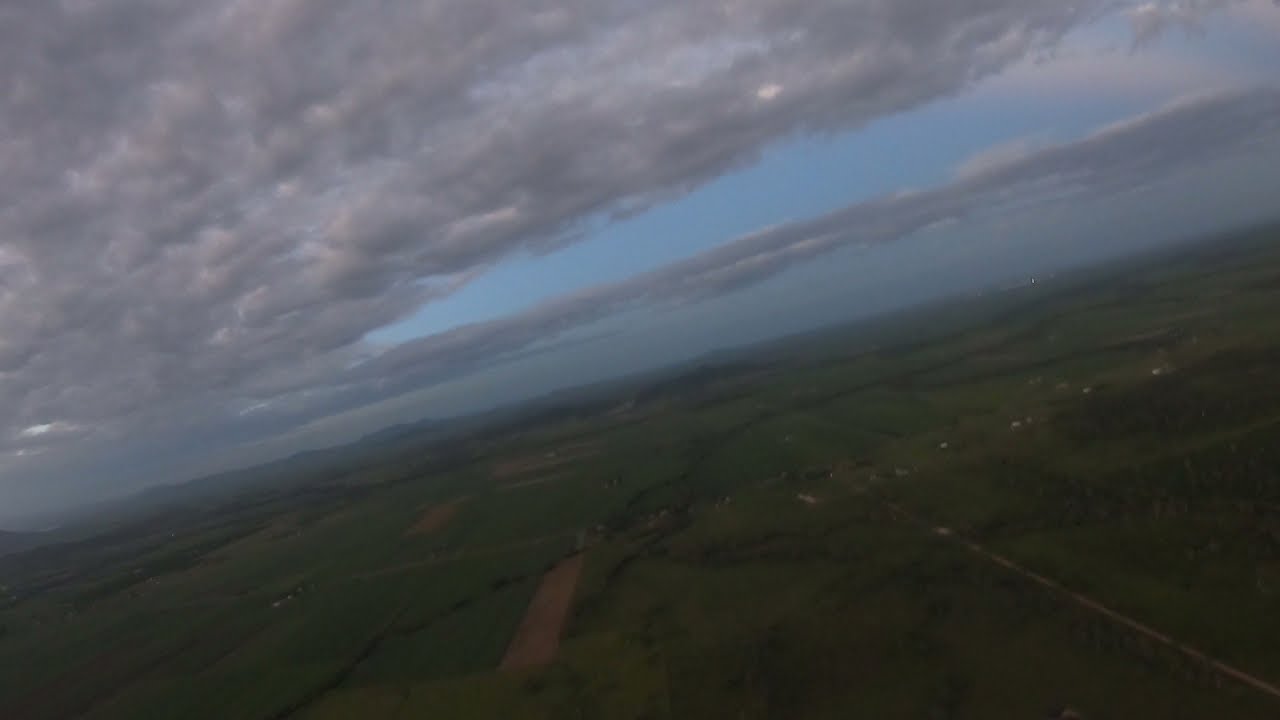This detailed aerial photograph, taken from either an airplane or a drone during the day, reveals a sweeping landscape below. The image has a slight tilt, so when viewed at a 45-degree angle, the orientation becomes clearer. The upper left-hand corner of the picture is dominated by a thick layer of gray stratus clouds, partially covering a sliver of pale blue sky. Below the cloud line, extending halfway down the image, a streak of gray haze can be seen.

The lower portion of the photograph showcases the terrain far below, comprised mainly of green fields interspersed with freshly tilled brown patches. From the midline on the right to a steeper angle downward on the left, a narrow dirt road lined with trees meanders through the scene. Sparse farmhouses are scattered across the landscape, with a few white buildings concentrated in the far right corner, suggesting a rural farmland area. Despite the predominantly overcast sky, it is evident that it is a clear day, allowing the vibrant natural colors of the landscape to be captured in rich detail.